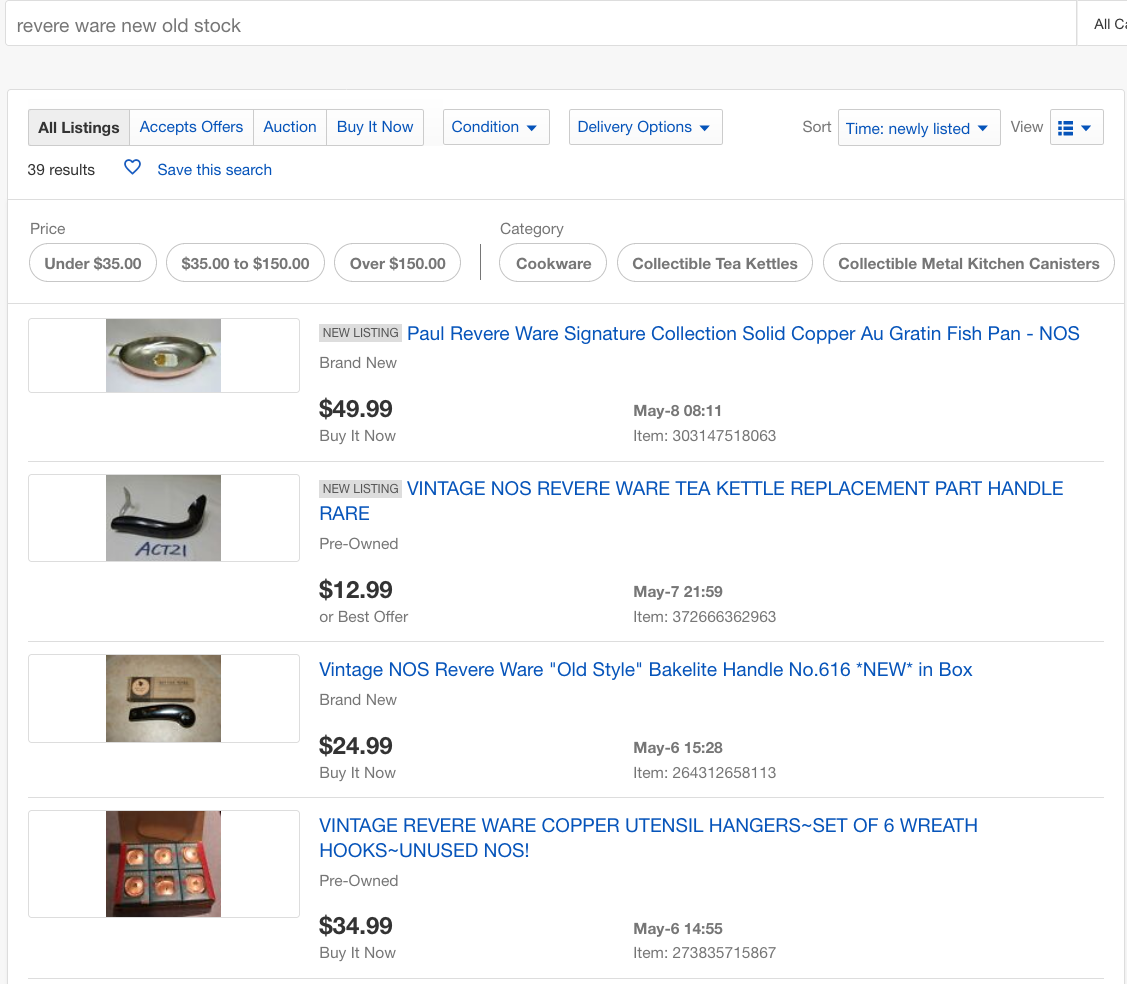The image displays a collection of vintage kitchenware items with their prices listed below. At the bottom, there's a vintage Revere copper utensil hanger set of six wreath hooks, tagged as unused and pre-owned, priced at $34.99 with a "Buy It Now" option dated May 6th, 1455. The item number is 273835715867. Next to the listing is a box containing several small copper items. Above this, there is a black device resembling an armrest but likely a handle replacement part, priced at $24.99. Another similar replacement part is listed for $12.99. Finally, there's a pan available for $49.99.